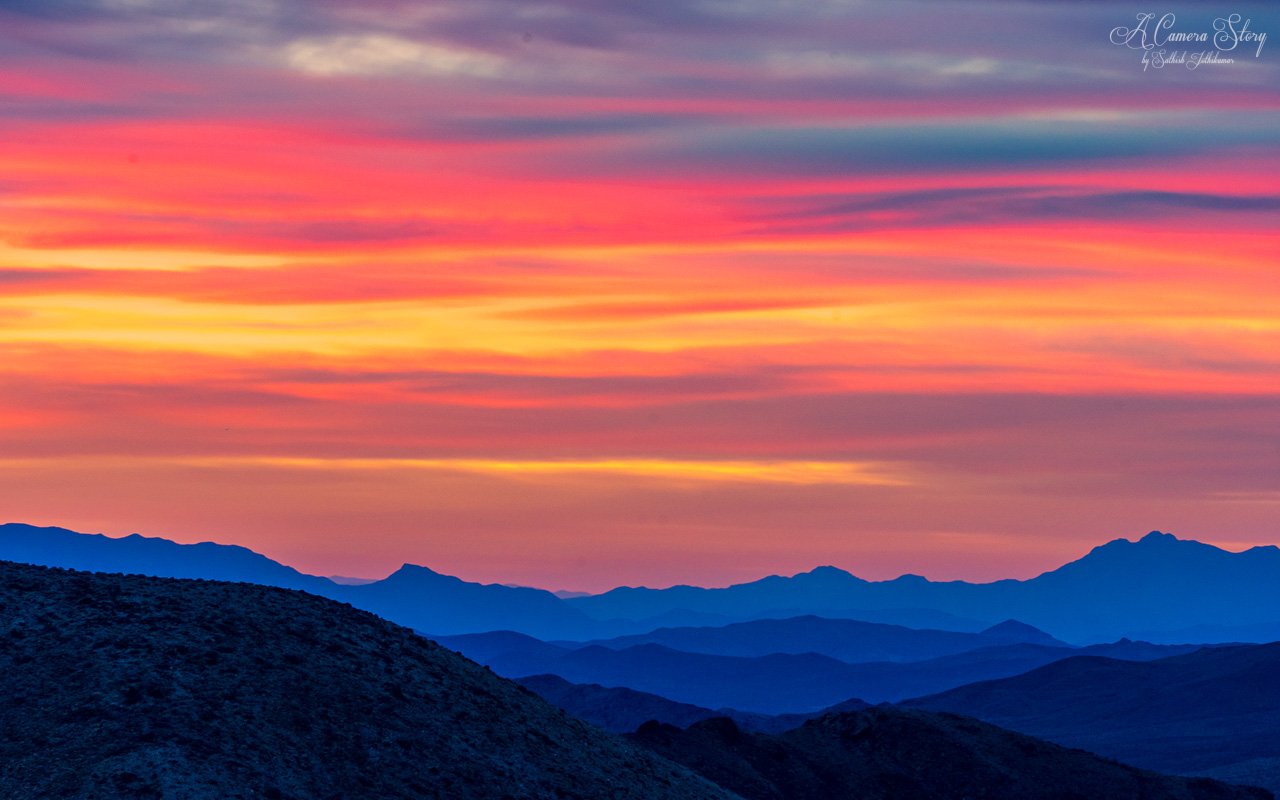A breathtaking landscape photograph captures an expansive view from a hillside, looking out over rolling hills and mountainous ranges into a striking sky at dusk. The sky occupies the top two-thirds of the frame, displaying a mesmerizing gradient that transitions through purples, reds, blues, oranges, and yellows. Darker clouds and the faint silhouette of a bird can be seen in the upper left corner, adding depth and intrigue. Below the vibrant sky, the silhouette of a mountain range stretches across the horizon, rendered in various shades of blue. The closer, foreground mountains are depicted in darker blue hues and slightly tinged with touches of green, suggesting grassy and dirt-covered terrain. On the left side, a small hill covered in grass and dirt slopes down towards the center, adding texture and balance to the composition. The image captures the serene and surreal beauty of nature at dusk with its harmonious blend of colors and contrasting silhouettes.